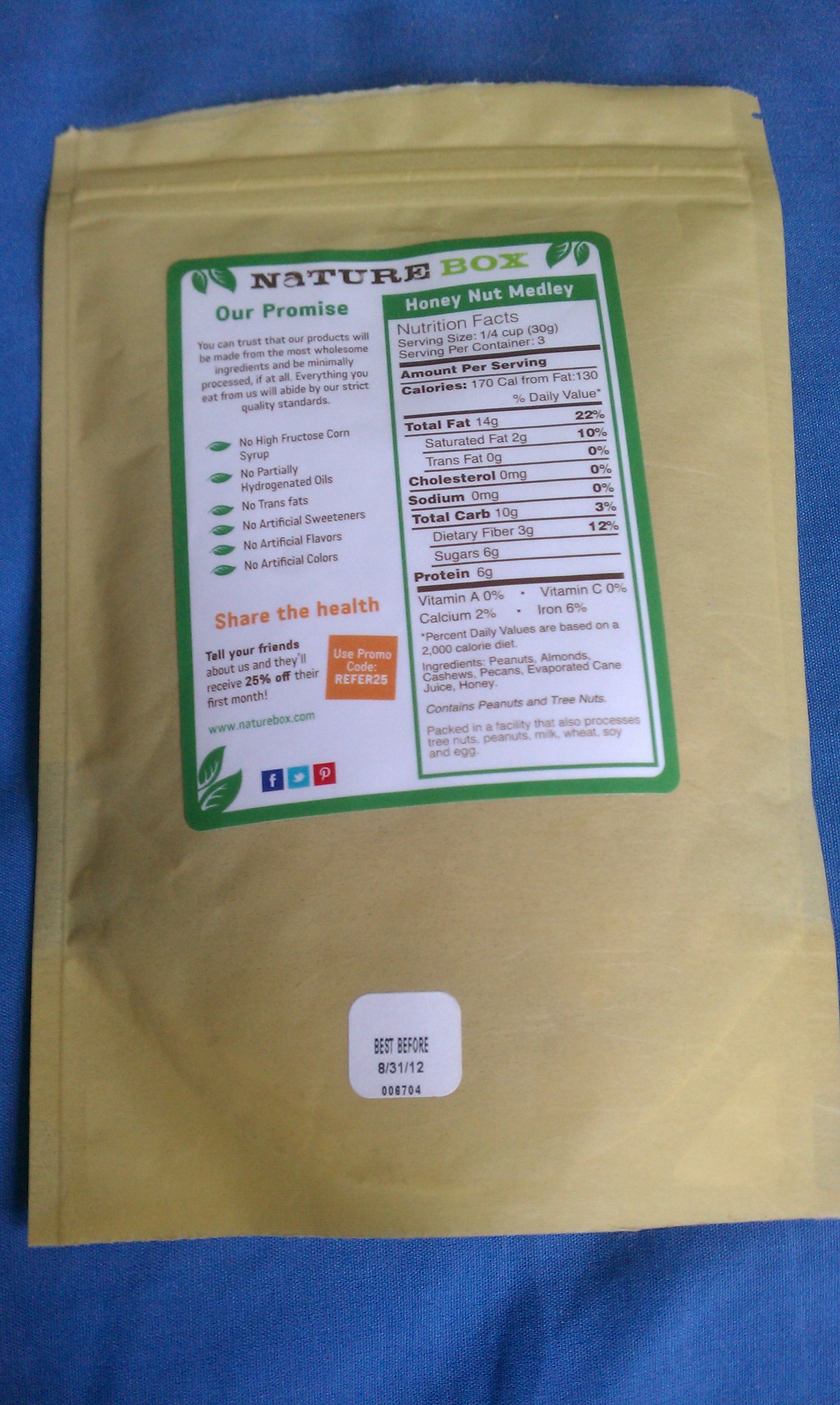This photograph features a package of nuts from Nature's Box, captured laying on a piece of blue fabric. The nuts are encased in a brown paper resealable bag, adding a rustic touch to the packaging. A small white sticker at the bottom of the bag indicates a "Best Before" date, reading "8-31-12." The main label, prominently displayed, identifies the product as "Nature's Box Honey Nut Medley." This label also includes various details about the company and its commitment to quality, the ingredients list, nutrition facts, and an orange square containing a promotional code. The text assures that the products are made from the most wholesome ingredients and are minimally processed, emphasizing the company's strict quality standards.